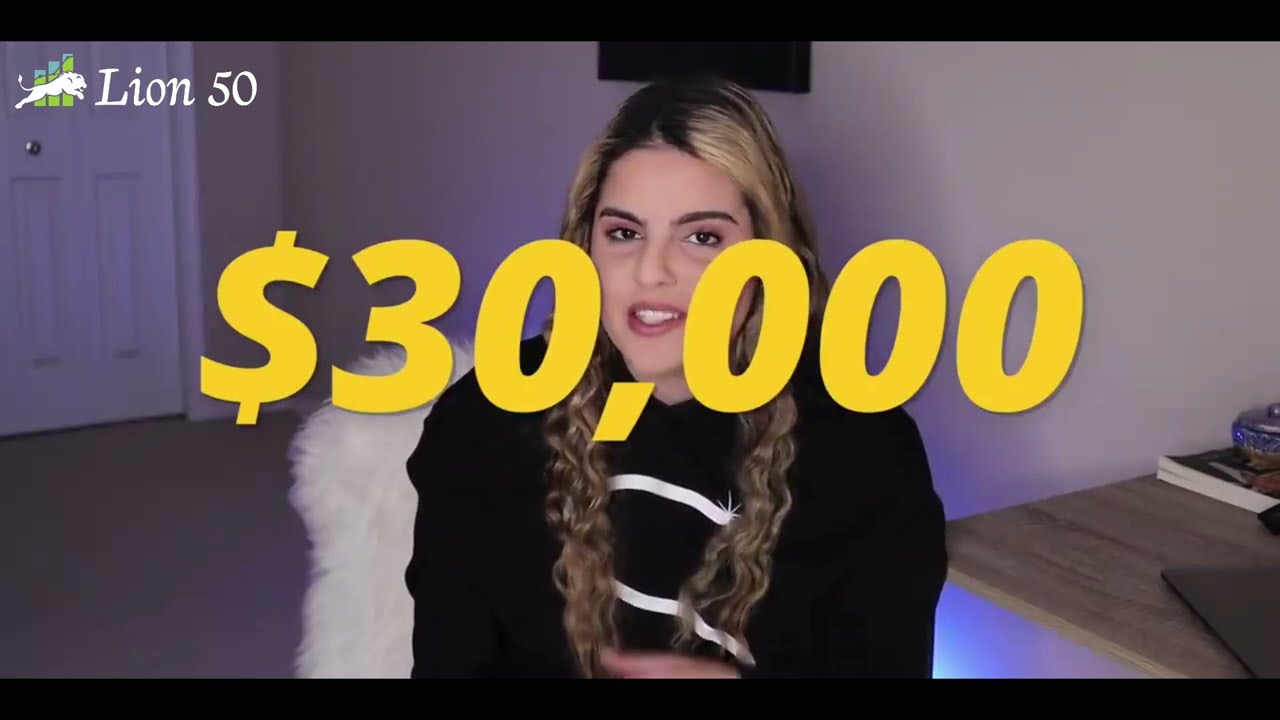In the image, a young woman with long, curly, blonde hair featuring black roots and twin braids cascading down her shoulders is seated in a chair with a fluffy, white, fur-like backing. She is wearing a black jacket or sweater adorned with white stripes across the chest. Prominently displayed in front of her is a bright yellow text that reads "$30,000." In the upper-left corner, there is a white lion logo jumping towards white text that reads "Lion 50." Behind the lion, three greenish bar charts progressively increase in height. To her right, mounted against the wall, is a light wood desk holding a stack of books and an open black laptop, bathed in a subtle purple and blue light from beneath the desk. The background features a white wall with a black TV screen descending halfway and a white door to the upper left. A thin black border frames the rectangular, wide-format image, reminiscent of a YouTube video screenshot.